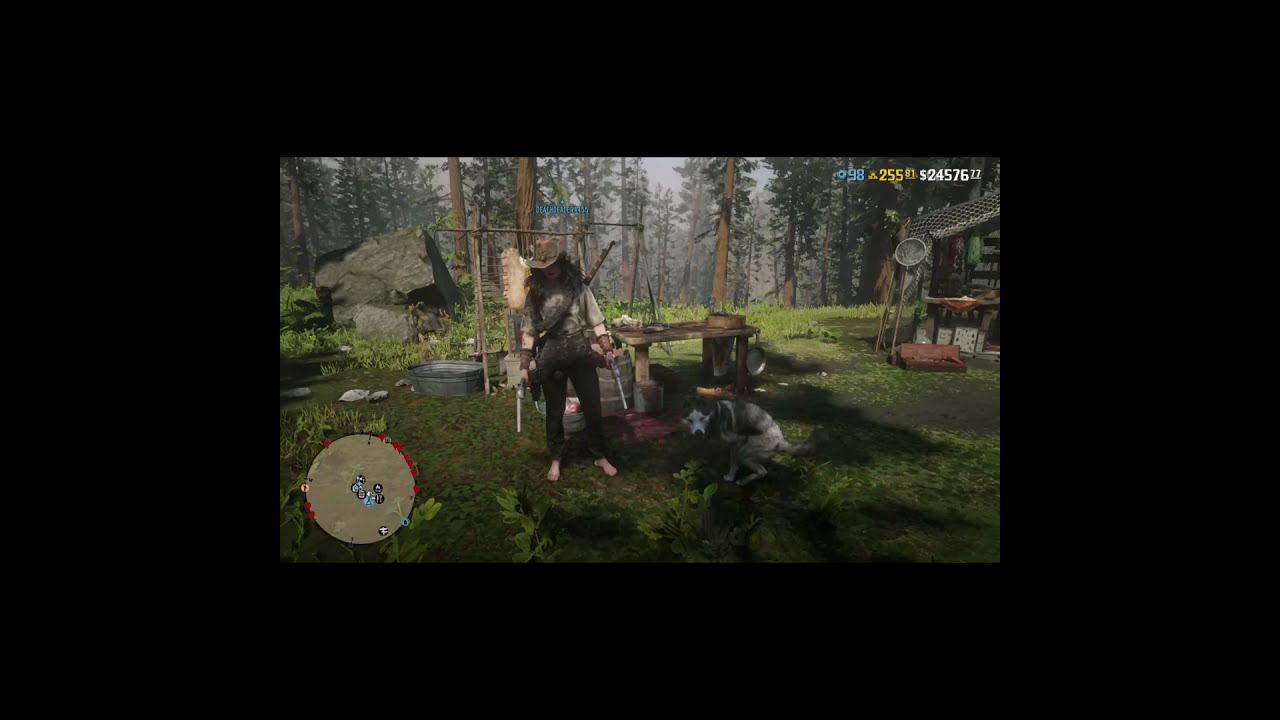This detailed caption combines the shared elements and distinct details from the three voice descriptions:

The image is a screenshot from a video game, likely with a setting similar to "Red Dead Redemption." It portrays a detailed outdoor scene in a dense forest filled with tall, brown trees topped with evergreen leaves. The central figure is a barefoot individual, possibly a woman, wearing long green pants and a matching green shirt. She dons a brown cowboy hat and has very long black hair. She stands confidently in the foreground, holding two guns, exuding a rugged, survivalist demeanor.

To the right of the woman stands a dog, squatting as if about to relieve itself, adding a touch of realism to the scene. The background reveals a makeshift camp area with a variety of elements that suggest a primitive, self-sufficient lifestyle. Behind her, slightly to the right, a small, rustic cabin or shack stands, likely a part of her settlement. A rough wooden table littered with items and various pails surround the scene, enhancing the aura of everyday life in the wilderness. There are also hints of a tannery area, a common sight in survival settings where one might skin animals.

An animal howls off to the left side of the image, deepening the wilderness atmosphere. The lower left corner of the screenshot features a circular game control interface, likely a map, while the upper right displays numerical values, possibly indicating game score, health, or stamina.

The colors dominate with greens and browns, complemented by deep reds, reinforcing the earthy, wild ambiance of the scene.